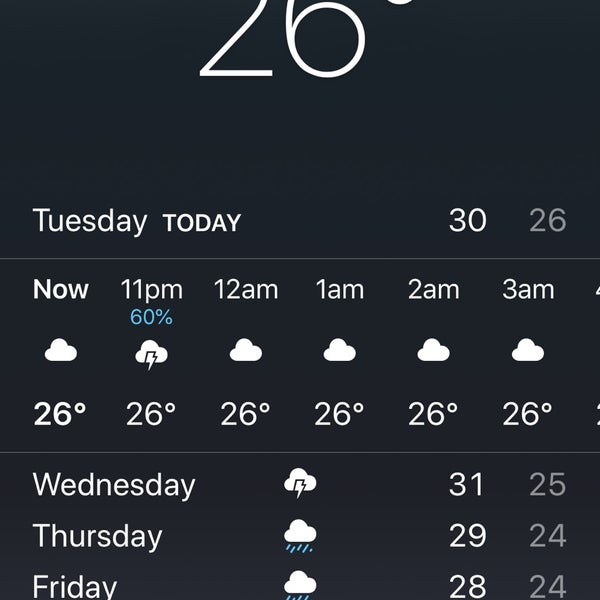Screenshot from the iPhone weather app, displaying the current weather conditions and forecast. The screen is slightly cut off at the top, but the temperature reads 26 degrees. Below, "Tuesday Today" is on the left, and on the right, it shows a high of 30 degrees and a low of 26 degrees.

The hourly forecast begins with "Now," showing 26 degrees, followed by "11 PM" with a 60% chance of precipitation accompanied by a cloud with a lightning bolt icon, indicating a thunderstorm and a temperature of 26 degrees. Subsequent hours, from "12 AM" through "3 AM," all show a temperature of 26 degrees with cloud icons.

Further down, "Wednesday" is noted with a cloud containing a lightning bolt, depicting thunderstorms, with temperatures ranging from a high of 31 degrees to a low of 25 degrees. For "Thursday," there is a cloud with rain coming out of it, indicating rain showers, with a high of 29 degrees and a low of 24 degrees.